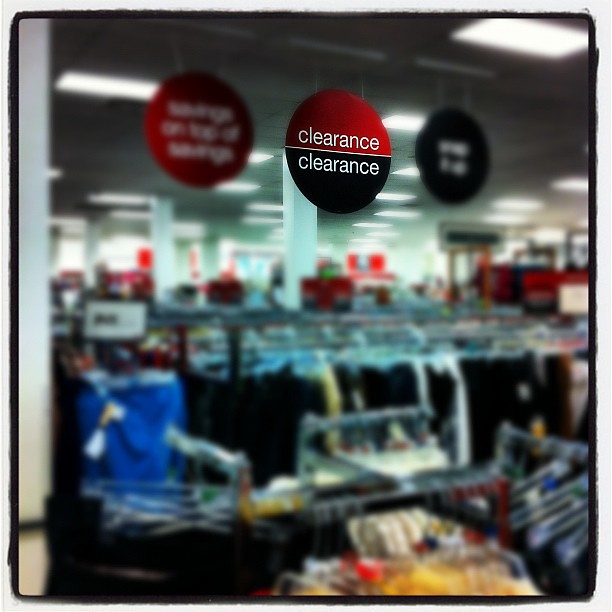The image depicts the interior of a retail store, specifically focusing on the clothing section. The store is filled with numerous racks, all brimming with various garments, creating a bustling and vibrant shopping environment. The photograph has been artfully edited to render everything slightly blurred, with the notable exception of a prominent sign positioned at the top center. This circular sign, which draws the viewer's attention, is clearly divided into two halves by a horizontal white line. The upper half of the sign is red, while the lower half is black, and both halves prominently feature the word "Clearance" in bold white letters. This sign indicates a sale or discounted section, adding to the attraction for potential shoppers. The overall ambiance of the image suggests a busy store environment with a focus on affordability.